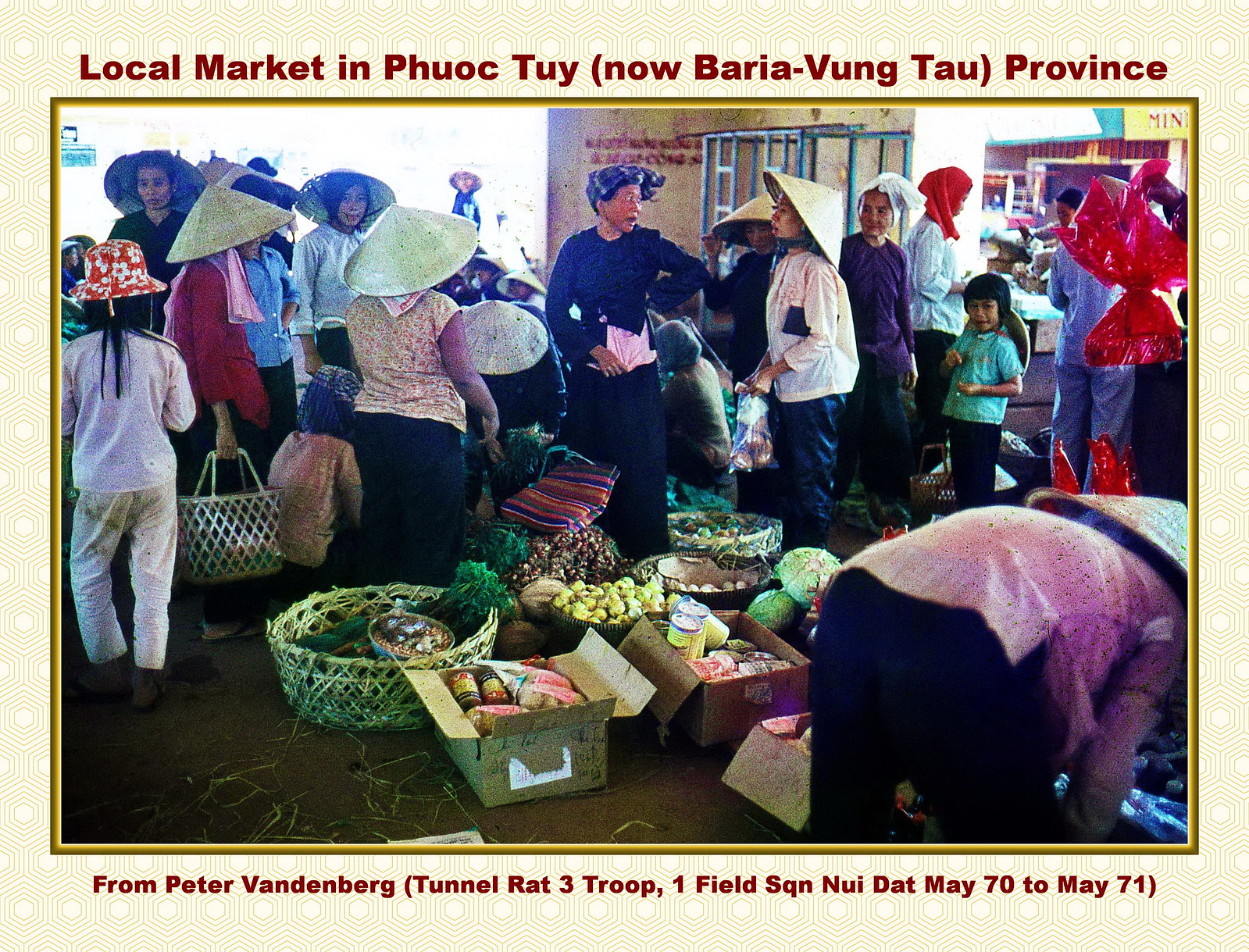The image is a wide rectangular photograph framed with a digital frame, which is narrower on the left and right sides and thicker at the top and bottom. The frame features a pattern of several repeating six-sided shapes bordered by similar shapes in yellow and slightly off-white hues.

At the top of the frame, in dark reddish-brown font, it reads: "Local market in Phuoc Tuy (now Baria Vung Tau province)." Below that, a caption says: "From Peter Vandenberg (Tunnel Rat 3 Troop, 1 Field Squadron, Nui Dat, May '70 to May '71)."

The color photograph depicts a bustling indoor-outdoor market scene in Vietnam, with several people, including many women and children, engaging in various activities. Most of the women are wearing traditional large conical hats. The market is filled with baskets of food, produce, canned goods, and other items. The women are dressed in colorful clothes, scarves, and blouses, predominantly wearing pants rather than skirts or dresses. Some are holding bags and other containers. A wall can be seen in the background, suggesting a transition to an outdoor space beyond.